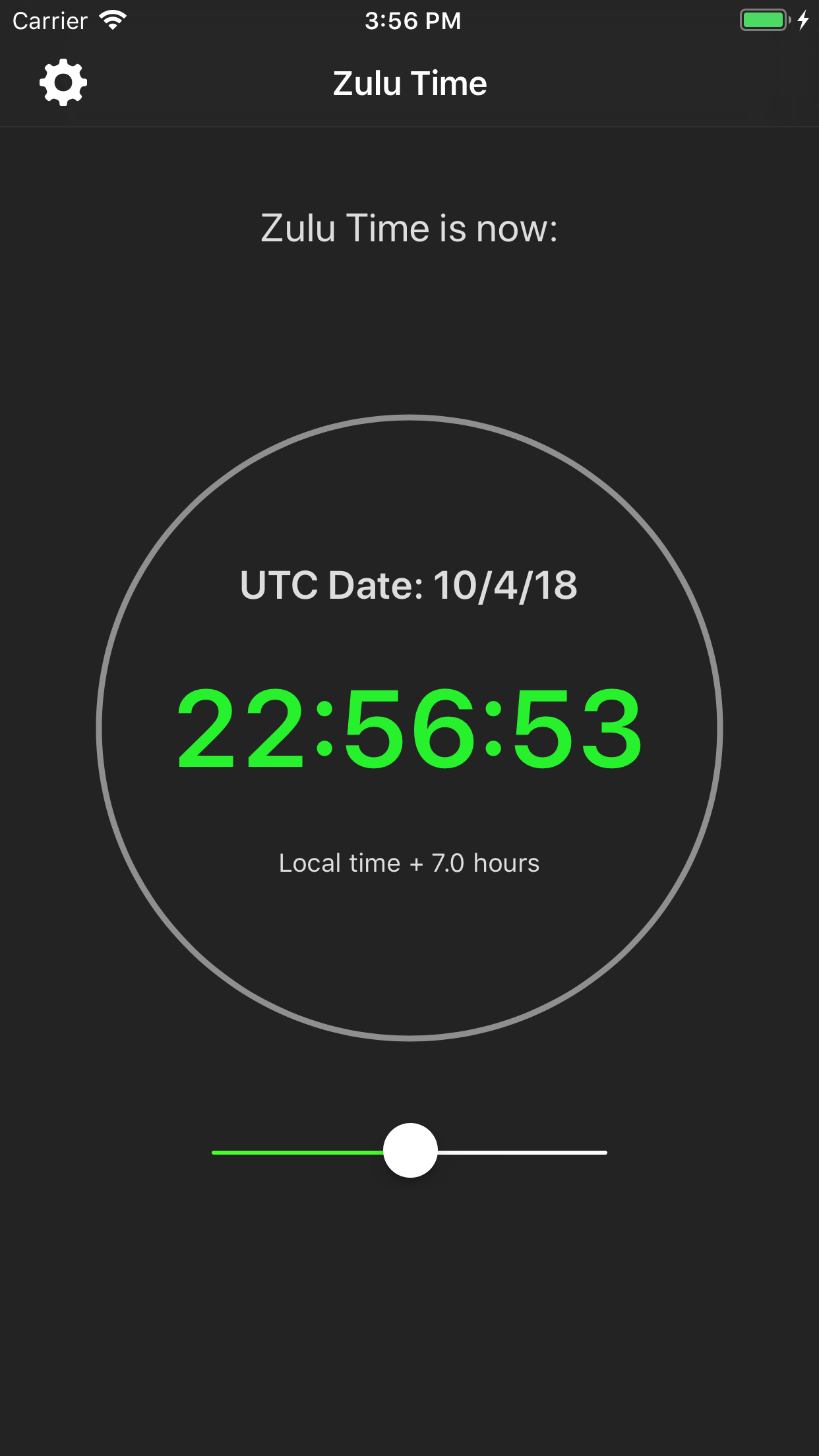This image is a screenshot captured from a mobile device. The top-left corner displays a generic label "Carrier" next to a Wi-Fi signal icon, indicating that the device is connected to a wireless network. The battery icon is fully charged. The top of the screen shows the time as 3:56 PM while the date is recorded as October 4, 2018. The device is set to Zulu Time (UTC +0), which is mentioned as being seven hours ahead of the local time shown. The time displayed prominently in the center of the screen is in military format reading 22:56:53, which converts to 10:56:53 PM in standard time. The background of the image is solid black, providing a stark contrast to the displayed text and icons.